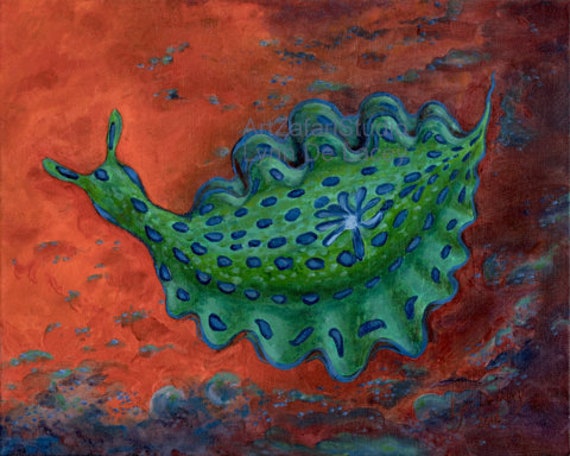The image is a highly stylized watercolor painting of a frilly snail-like sea creature, set against a vibrant red and orange oceanic background with hints of green and blue, suggestive of coral. The snail's body is predominantly green with intricate blue patterns, and it features scalloped wings or fins edged in blue. Its head sports tentacle-like ears, adding to its whimsical appearance. The creature also has a distinctive blue flower with a white center on its back, making it appear almost otherworldly. Gray billows or puffs add a dreamy, nearly smoky effect to the composition, which is reminiscent of illustrations found in children's books.